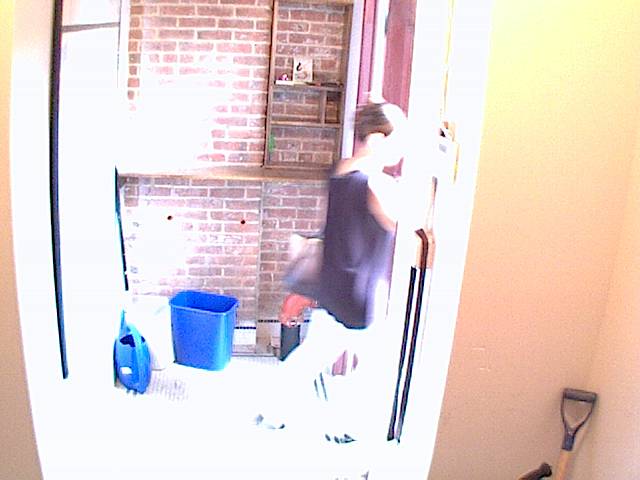In this bright and somewhat blurry indoor photograph, a noticeable glare from sunlight casts a white light over the scene. A woman, wearing white pants and a purple sleeveless top, walks out of a door with a purple frame. This door is centrally right, with a security alarm attached to the wall nearby. The room features a red brick wall adorned with wooden shelves, one of which holds a picture, while the others remain empty. In the foreground at floor level, a blue wastebasket and a blue watering can for plants are visible. Additionally, the upper part of a shovel with a natural wood handle is partially seen in the right corner of the frame. The walls of the room are a yellow-brown, adding a warm hue to the interior.